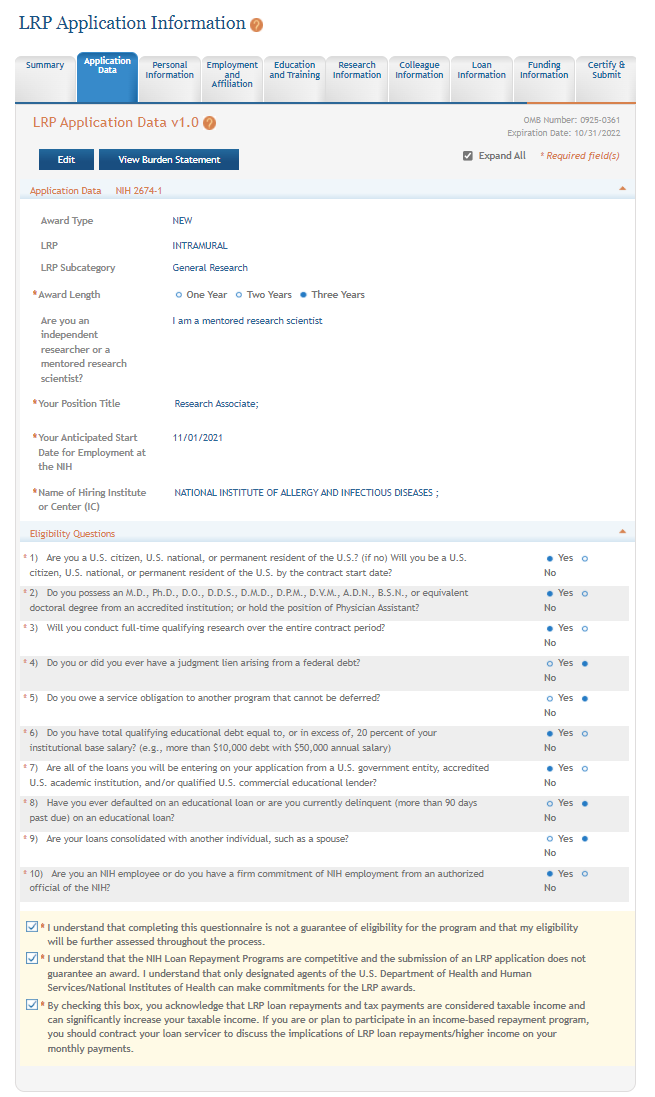The image depicts a detailed web page for an LRP (Loan Repayment Program) application. At the top, prominently displayed, is the heading "LRP Application Information." The interface contains various navigation tabs, including Summary, Application Data, Personal Information, Employment and Affiliation, Education and Training, Research Information, Colleague Information, Loan Information, Funding Information, and Certify and Submit.

In the top right corner, an OMB (Office of Management and Budget) number, 0925-0361, is noted with an expiration date of 10-31-2022. Highlighted in orange text is the title "LRP Application Data v1.0." Two blue buttons are visible: one labeled "Edit" and another labeled "View Burden Statement."

Further down, the section titled "Application Data" features a form identified as "NIH 2674." Under "Award Type," it specifies "New" and "Intramural." This is followed by several subcategories, including "LRP Subcategory" and "Award Length," with options for 1 year, 2 years, or 3 years, the last of which is selected.

A question asks, "Are you an Independent Researcher or a Mentored Research Scientist?" The response indicates, "I am a Mentored Research Scientist," with the position title of "Research Associate." The anticipated start date is noted as 11-01-21. The hiring institute or center is identified as the National Institute of Allergy and Infectious Disease (NIAID).

There are ten eligibility questions listed in black text on a gray and white background. At the bottom of the page, there are three checkboxes for different informational declarations. The overall appearance of the page is that of a comprehensive application form, meticulously organized and detailed.